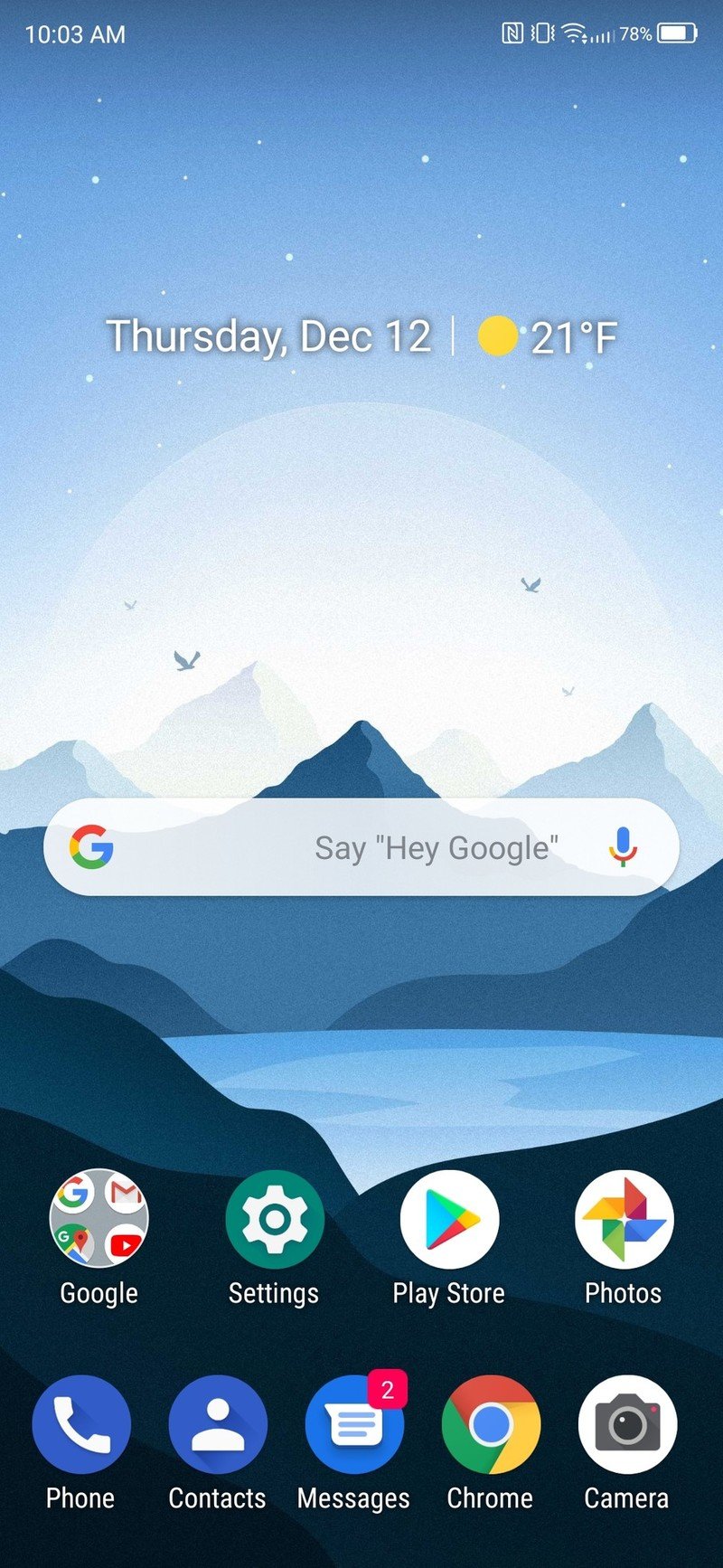The image portrays a smartphone screen capturing a picturesque landscape. The upper part of the screen displays key information: the time is 10:03 AM, there is good internet reception, and the battery is at 78%. The background image is reminiscent of a northern region, possibly Alaska, featuring rolling hills in the foreground, a serene bay, and snow-capped peaks in the distance. Above the majestic mountains, the sky transitions from light blue to a deeper hue, almost venturing into space, with the sun brightly shining behind the peaks.

In prominent white text, the screen indicates it is Thursday, December 12th, with the current temperature being a chilly 21 degrees Fahrenheit under sunny skies. A Google search bar appears beneath this, offering the option for voice search via a microphone icon or the "Hey, Google" command.

The bottom section of the screen is populated with app icons: Google, Settings, Google Play Store, and Google Photos. Further below, a navigation bar features essential applications: Phone, Contacts, Messages (indicating two unread messages), Google Chrome, and Camera.